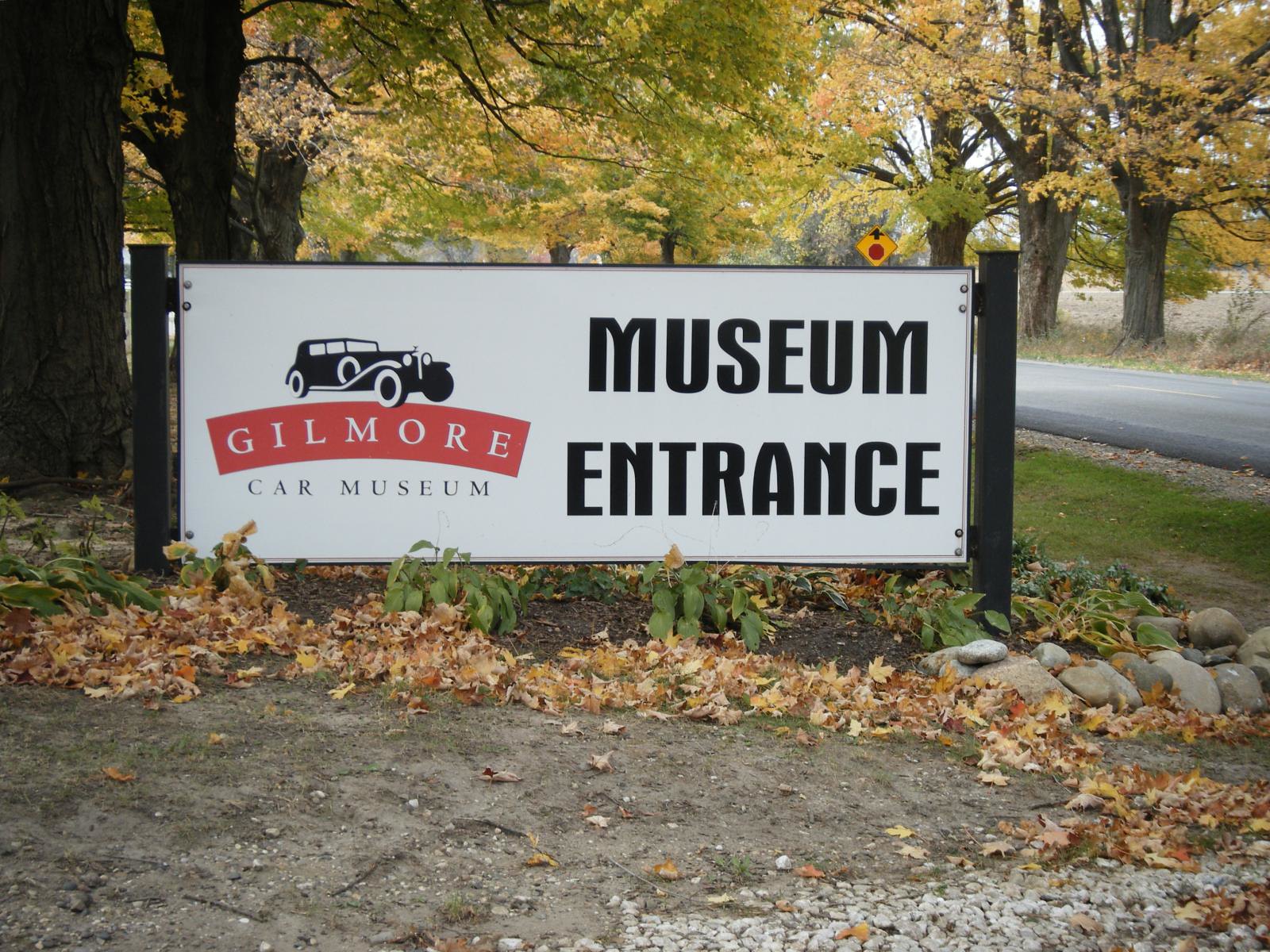A full-color photograph captures an autumn scene outside, marked by trees with leaves in various stages of changing color and numerous fallen leaves scattered on the ground. Prominently displayed in the center is a large white wooden sign mounted on two black metal posts. The sign features an image of an antique car to the left, beneath which a red banner displays the word "Gilmore" in white text. Below the banner, "Car Museum" is written in black text, and to the right, large black letters announce "Museum Entrance." Surrounding the sign are rocks, some green plants, and a dirt pathway. On the right side of the image, a road is visible along with a yellow diamond-shaped street sign indicating an upcoming stop sign. The sky in the background peeks through the trees, adding to the rural charm of the scene. There are no people or animals present in the photograph.